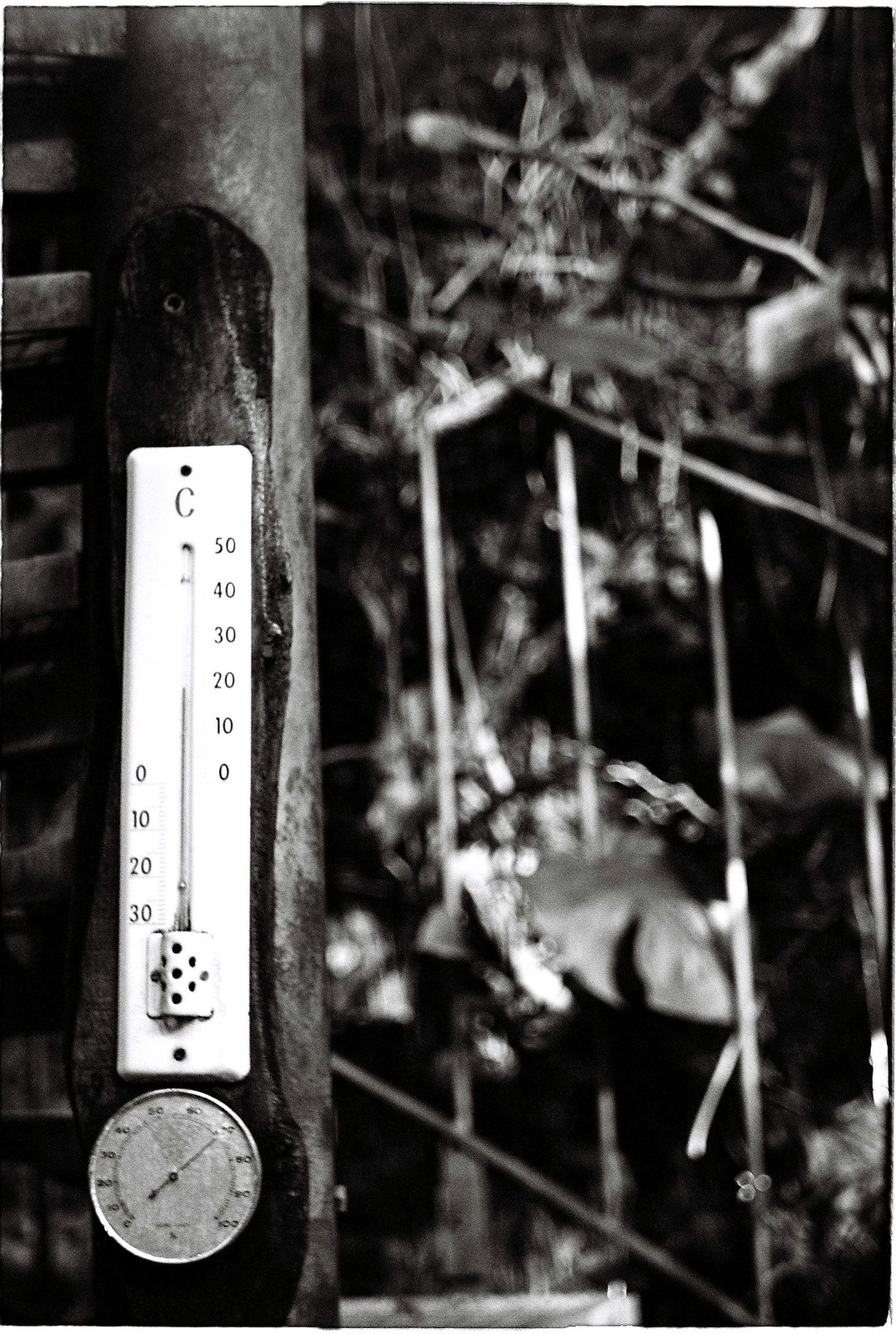A black-and-white photograph showcasing a vertical white thermometer and a dial hygrometer attached to a square wooden post, possibly a part of a cabin's banister. The thermometer at the top prominently displays a large "C" for Celsius, with temperature markings on the right side descending from 50 to 0 degrees, and on the left side ascending from 0 to 30 degrees, indicating both above and below freezing temperatures. The mercury in the thermometer reads just below 20 degrees Celsius. Below the thermometer, the dial hygrometer measures humidity. In the background, a metal railing for a small staircase is visible, along with various plants and leaves protruding through the banister rails. Wooden planks are also attached to the left side of the post, adding to the rustic charm of the scene.